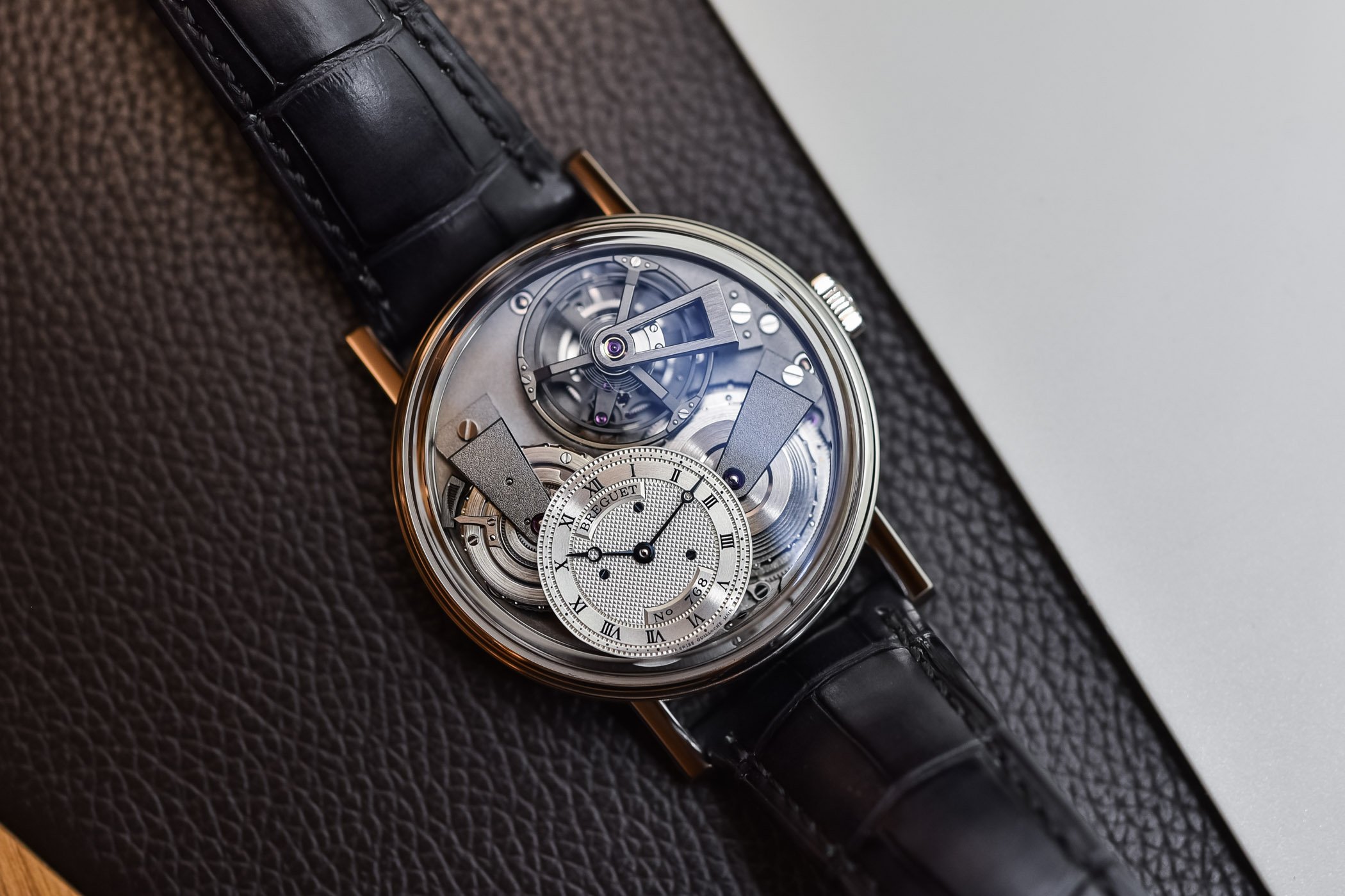This image features a stunning, intricately designed mechanical watch in a close-up, horizontal composition. The watch, positioned on a piece of black leather that rests atop a brown wooden surface with a gray wall in the background, showcases a captivating blend of artistry and engineering. Encased in a shiny silver metal, the circular watch face is partially transparent, revealing a mesmerizing array of gears and mechanisms that give it a highly technical and elaborate appearance.

On the lower-left portion of the watch face, there is a smaller silver dial that displays the time using Roman numerals, with elegant black hands ending in small circles. A silver crown protrudes from the right side, allowing adjustments to the time. The overall color scheme of the watch face includes dark blue-gray tones and additional silver highlights, with a notable purple jewel embedded in the upper section, reminiscent of the motor that powers the intricate movements.

The watch's black leather strap adds a touch of sophistication and comfort, complementing the luxurious and refined look of the timepiece. The detailed construction and visible mechanical components suggest that it is a meticulously crafted, high-end watch, made with great expertise and precision.